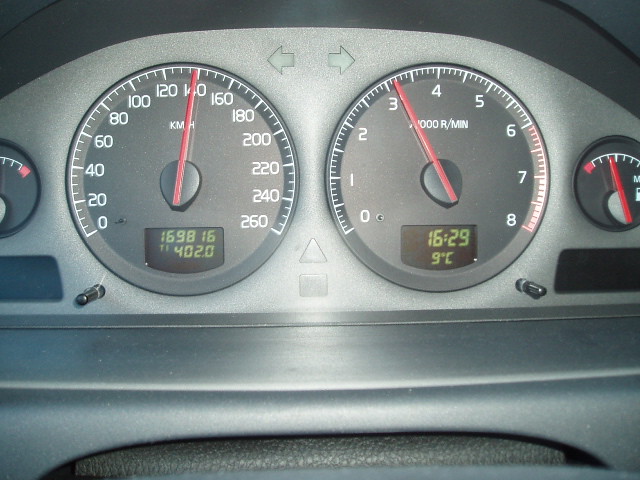The image depicts the dashboard of a typical sedan, showcasing a variety of meters and digital readouts. There are four primary gauges visible beneath the dashboard, although only three are clearly discernible. One of these gauges appears to be for temperature but is partially obscured. The fuel gauge indicates a little over half a tank, while the RPM gauge shows that the engine is running slightly above 3,000 RPMs. 

Additionally, there are digital readouts including a clock and a thermometer. The clock displays 16:29, which equates to 4:29 PM, and the thermometer shows a temperature of 9 degrees Celsius. The speedometer reads 140 kilometers per hour and the car's odometer shows a total distance of 169,816 kilometers traveled, with the current trip log at 402 kilometers. These digital readouts display important information such as total mileage and time/temperature readings.

Daylight is clearly visible, illuminating the dashboard and causing a slight glare off the surfaces around the gauges. Overall, the car has the characteristics of a standard sedan, providing essential driving information in a clear and organized manner.